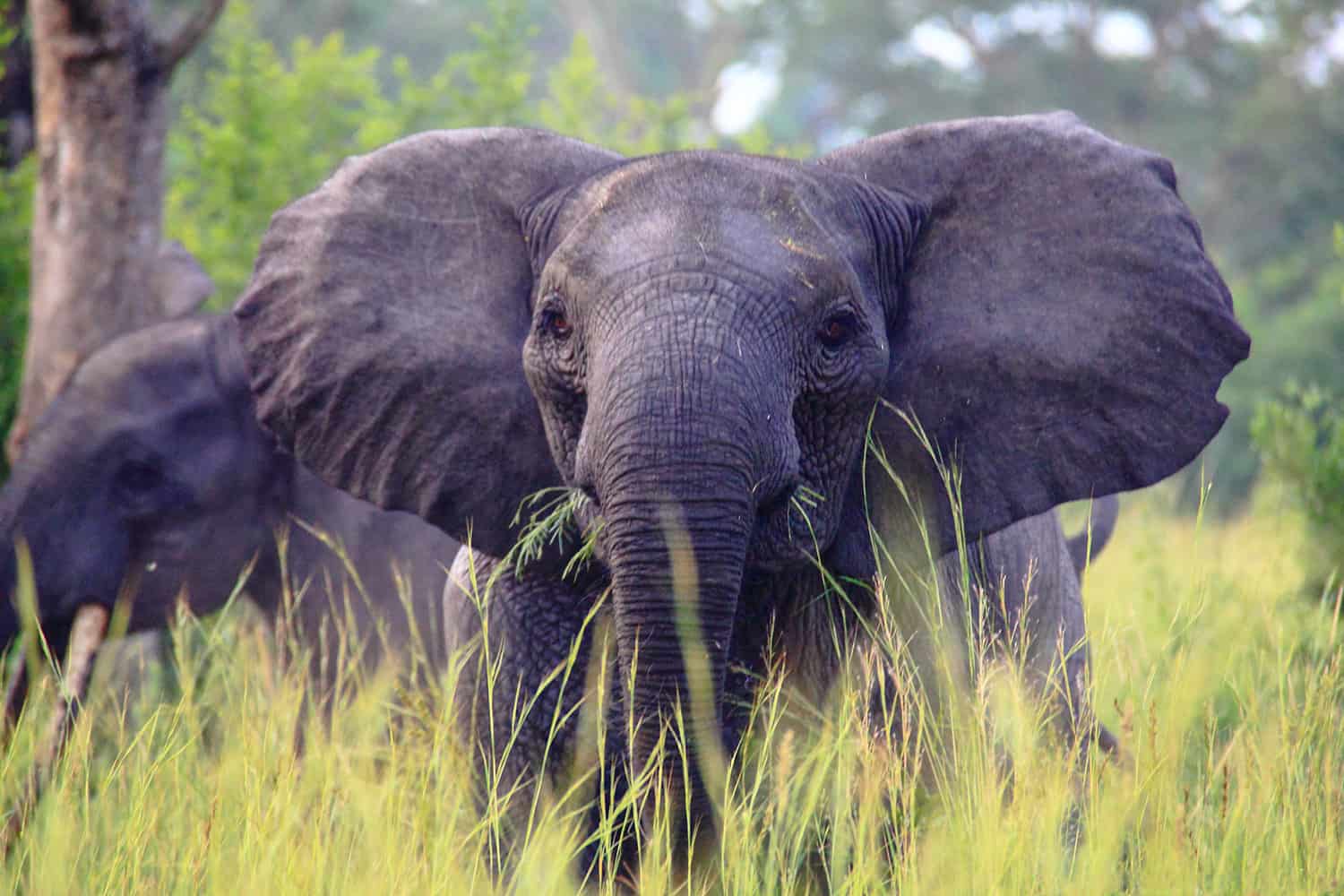The image captures a baby elephant standing amidst tall, wild grass, which partially obscures the lower part of its body. The baby elephant, distinguished by its smaller size and absence of tusks, is engaged in eating grass, with its trunk actively foraging. Its ears, characteristic of a young elephant, are not as large as those of an adult. Behind this young elephant is another, larger elephant, adding context to the scale and size of the baby. The background features a blurred forest, enhancing the focus on the elephants in the foreground. The tall grass and some visible tree trunks along with oversized wild plants contribute to the rich, natural habitat in which these elephants reside. The baby elephant’s skin showcases different shades of gray, with noticeable lines on its trunk and under its eyes, hinting at the intricate details of its youthful features.